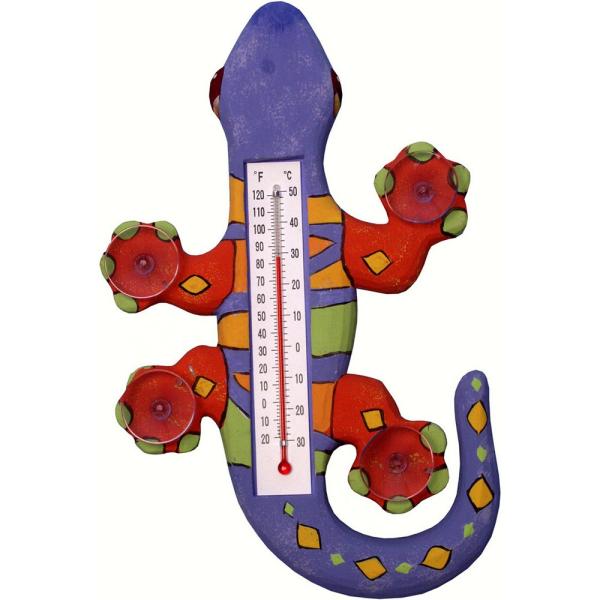The image displays a decorative thermometer encased in an artistic representation of a gecko, vertically aligned against a solid white background. The thermometer itself features markings for both Celsius (°C) on the left and Fahrenheit (°F) on the right. The Celsius range spans from -30 to 50 degrees, while the Fahrenheit range goes from -20 to 120 degrees, with a red mercury bar indicating a current temperature of approximately 25°C (78°F). 

The gecko design includes a suction cup at the top, used for attachment to a surface like glass. The gecko's head is light blue with black eyes, facing upward. The body, decorated with colorful stripes of yellow, orange, green, and light blue, transitions into a long tail that curves to the right and upward, detailed with alternating green and yellow diamond-shaped patterns. The limbs are orange with green fingertips. The overall look merges functionality with a playful artistic aesthetic, combining practical use with decorative flair.